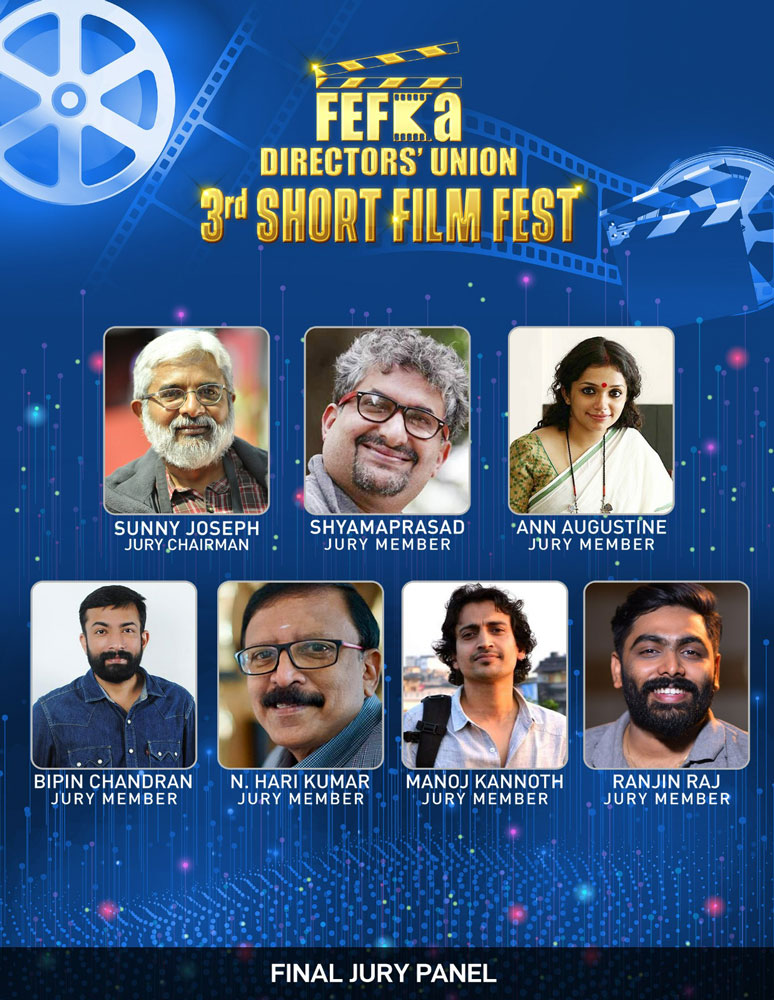This promotional image, designed as an infographic, highlights the final jury panel for the FEFA Directors Union Third Short Film Fest against a predominantly blue background adorned with 3D graphics of film reels, film strips, and a director's clapboard. At the very top, gold text prominently announces "F.E.F.A. Directors Union Third Short Film Fest." The image is split into two rows featuring photographs and names of the jury members. The top row consists of three photographs: Sonny Joseph, an older man with a white beard and mustache labeled as the Jury Chairman, alongside Shyam Prasad and Ann Augustine, both identified as Jury Members. The bottom row displays four photographs with corresponding names: Bipin Chandran, N. Hari Kumar, Manoj Kanoff, and Ranjan Raj, each listed as Jury Members. At the very bottom, a semi-transparent black banner with white text reads "Final Jury Panel," signifying the collective role of these individuals in the film festival's judging process.